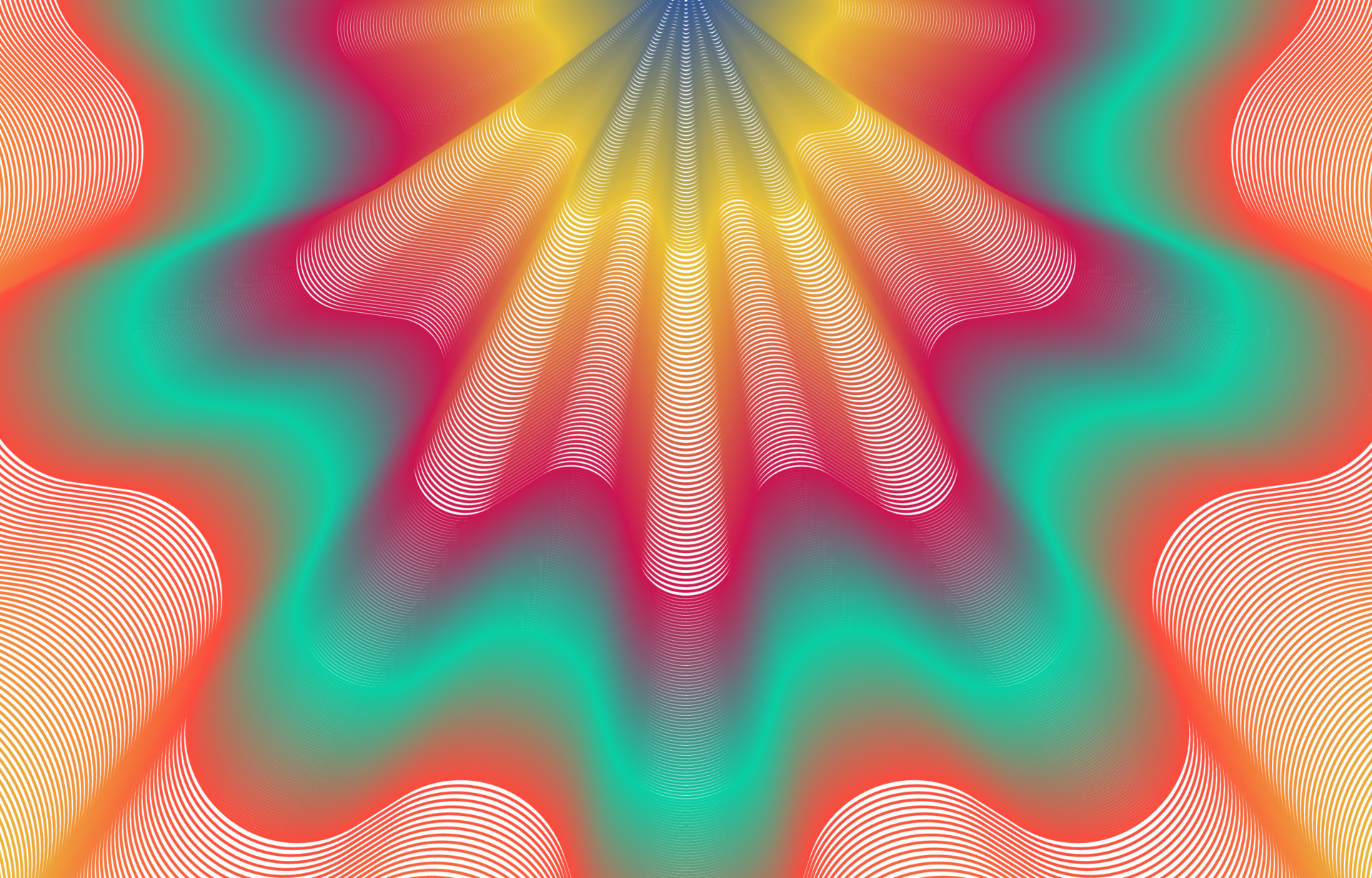This abstract artwork, which appears to be computer-generated, features an intricate, undulating pattern reminiscent of squiggly or fluted lines that evoke the appearance of a seashell or clamshell design. The image is rendered in vibrant, neon colors and spans a long, narrow horizontal frame. The eye is drawn to the center top where a bluish-gray hue begins and unfolds into a spectrum of colors including yellow, pink, and red that descend towards the bottom. This central pattern, resembling a teepee or the peak of an extended fabric, expands outward in flowing, wavy lines with a melting effect into green and orange at the edges. The outer borders are framed with stripes of reddish-orange and occasional yellow shades, providing a dynamic and psychedelic visual experience. The blending of the colors—ranging from cool turquoise and bluish-greens to warm oranges and reds—creates a cohesive and mesmerizing artistic piece that almost seems to move or rotate when gazed at for an extended period.